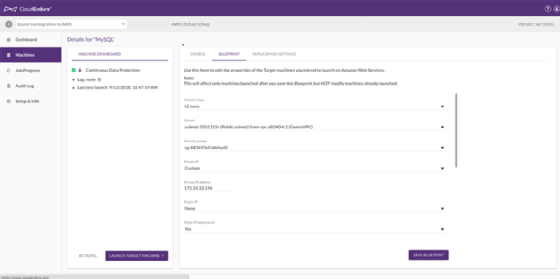In the image titled "Cloud Couture" (or a similar name), the text is very small and hard to read, but here is a detailed description of the layout. At the top of the page, there is a purple banner bar. In the top-right corner of this bar, a question mark icon serves as a help feature, and next to it, there is another logo for a different function. Below the banner bar, a drop-down box is visible, though its details are unclear.

On the left-hand side of the page, there is a vertical menu featuring several options. The top option is labeled 'Dashboard,' followed by four other clickable options. The second option in this menu is highlighted in purple. Immediately next to this vertical menu, there is a box labeled "Details for MySQL," which seems to be related to coding. Inside this box, there are three smaller options, one of which is marked by a green dot or check mark, though it's difficult to discern clearly. At the bottom of this box are a white 'Actions' button and a purple button labeled "Launch Target..."

To the right of this section, taking up the majority of the space, is a larger box with approximately six drop-down menus. Embedded within the fifth line of this section is a version or serial number, but it's hard to read due to the small font size. This intricate layout appears to be part of a user interface, possibly for a coding or cloud management platform.